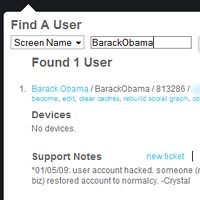The image appears to be a small screenshot of a user interface, likely from an administrative control panel, possibly from a platform like Twitter. The background is black with a white square overlay, giving it a dialogue box appearance. In the upper left corner, gray text reads "find a user" beside a drop-down menu where "screen name" is selected. To the right, in a search box, "Barack Obama" is typed in black letters. Below, gray text indicates "found one user," followed by "1" in black, and a light blue listing: "Barack Obama / Barack Obama / 813286". Additional menu items include "devices" (with "no devices" noted below), "support notes," and to the right, a light blue "new ticket" option. At the bottom, black text details an incident: "01/05/09 user account hack, someone restored account to normalcy - crystal."